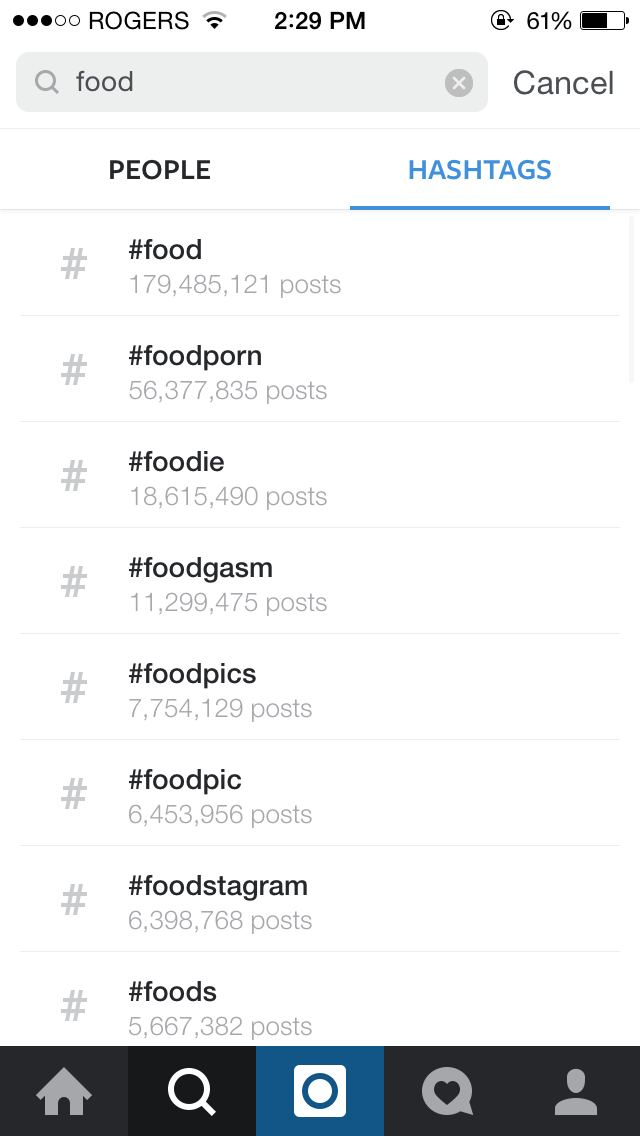The image depicts a screenshot from a mobile device, showcasing a search feature within an application, likely an older version of Instagram. At the very top of the screen, the device status display reveals the network carrier as "ROGERS" in all capitals, with three black circles and two white circles. The Wi-Fi signal strength indicates two out of three bars. The time shown is 2:29 p.m., the device is locked, and the battery is at 61%.

Below the status bar is a search box labeled "food" accompanied by a magnifying glass icon and an option to exit or cancel the search.

The content beneath the search box consists of two columns: "People" and "Hashtags." However, only the "Hashtags" column is visible. The following hashtags are listed alongside the number of associated posts:
- #food: 179,485,121 posts
- #foodporn: 56,377,835 posts
- #foodie: 18,615,490 posts
- #foodgasm: 11,299,475 posts
- #foodpix: 7,754,129 posts
- #foodpik: 6,453,956 posts
- #foodstagram: 6,398,768 posts
- #foods: 5,667,382 posts

At the bottom of the screen, there is a navigation bar with icons displayed in whitish-gray on black, including:
- A house icon
- A magnifying glass icon
- An icon resembling the Instagram logo, though less colorful
- A text bubble with a heart inside
- A person icon

Overall, this screenshot provides a detailed view of a user exploring popular food-related hashtags within the app, suggesting the interface and options available within this older version of the platform.